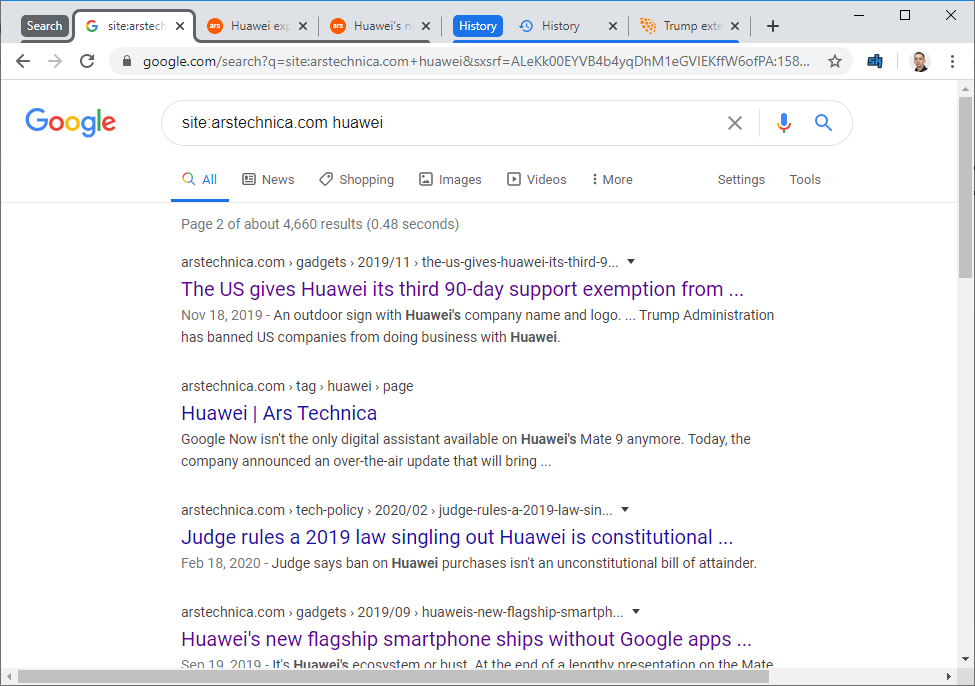In the upper left corner of the web page, there's a small black square labeled "Search" in white text. Five tabs are open at the top of the browser. The active tab is Google, displaying the search query "site:arstechnica.com Huawei," though some of the text is cut off. The second and third tabs both feature the Huawei logo in orange. The fourth tab is blue with a white clock icon and the word "History." The fifth tab shows part of a word, "Trump," and seems to depict a wing-like image. To the right of the tabs, the browser interface shows the symbols for minimize, full screen, and close.

Below the tabs, there are backward and forward navigation arrows, with the forward arrow grayed out, indicating it hasn't been used. Next to these is the reload icon, followed by the address bar. The URL in the address bar reads "google.com/search?q=site%3Arstechnica.com+Huawei…" but is truncated. There's a padlock icon indicating a secure connection, and a star icon for bookmarking.

Two more tabs are present, one blue and one with a face icon, though their details aren't clear. On the Google search results page, the query being searched is "site:arstechnica.com Huawei." The microphone icon for voice search is visible next to the search bar.

Below this are the Google search categories: All, News, Shopping, Images, Videos, More, Settings, Tools, with "All" currently selected. The search results indicate page 2 of about 4,660 results, found in 0.48 seconds.

The visible search results include four entries:
1. A listing about the US giving Huawei its third 90-day support exemption dated November 18, 2019. The headline is cut off.
2. A second entry from Ars Technica discussing Huawei's Mate 9 digital assistant update.
3. A third entry about a judge ruling on the constitutionality of a 2019 law affecting Huawei, dated February 18, 2020.
4. A fourth entry about Huawei's new flagship smartphone shipping without Google apps, dated September 19, 2019.

Overall, the image captures a detailed snapshot of a web browser displaying a focused Google search on Huawei and Ars Technica, highlighting the browser interface and search results.